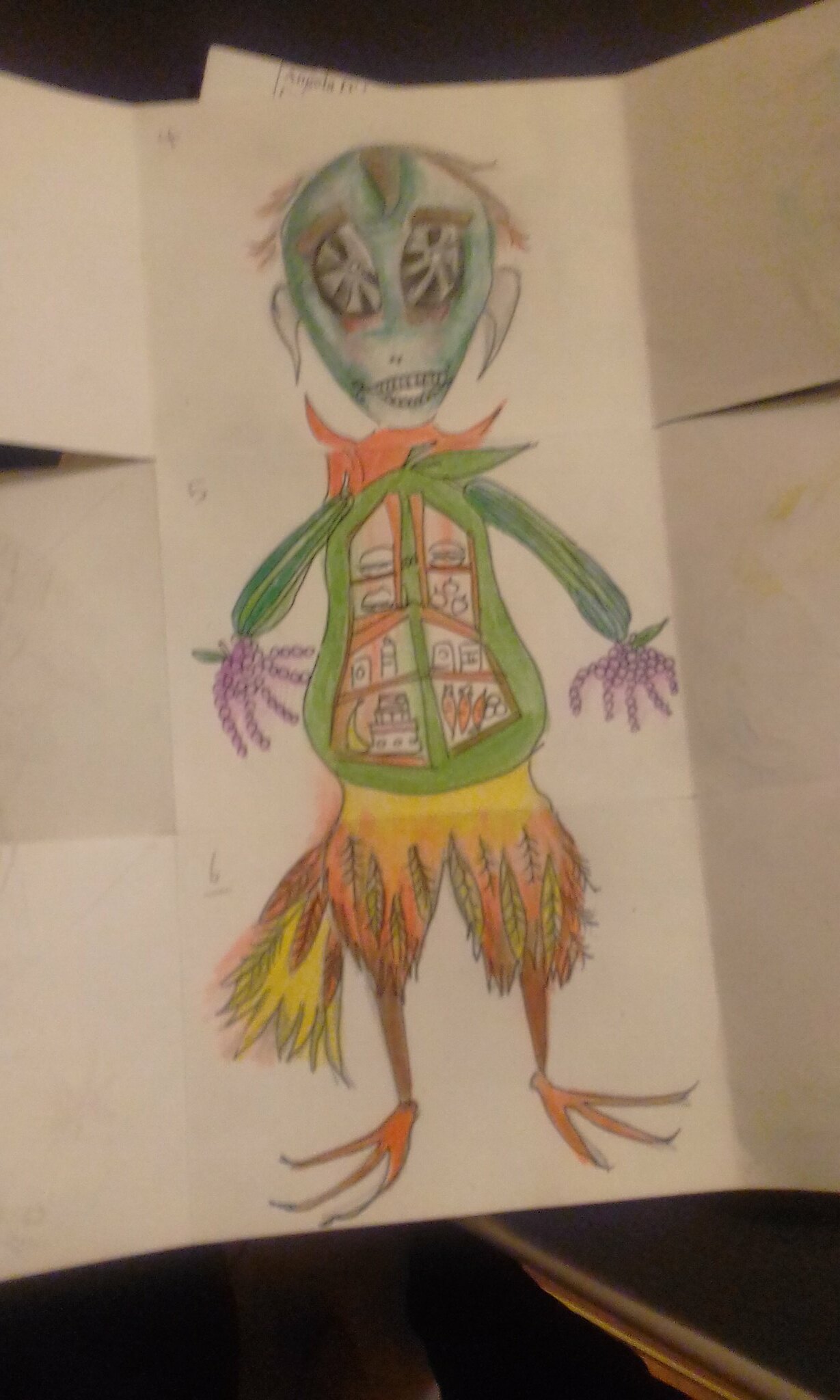This image showcases a photographed illustration spanning three sections of trifold paper, intricately assembled to form a bizarre creature. Each rectangular paper section contributes a unique part to the composite drawing. 

Starting from the bottom, the third section features a feathery lower body with gangly, claw-like legs reminiscent of distorted chicken feet. The number "6" is penciled in the top left corner.

The middle section, numbered "5," depicts the creature's pear-shaped, green torso. The torso is intriguingly designed to resemble a cupboard with glass windows, displaying various objects such as a banana and several bottles. The creature's arms extend from the torso, resembling green pickles, with fingers that look like grapes.

The top section, presumably labeled "4," portrays an alien-like blue head adorned with large black eyes encased in coral-like rims, tufts of hair, and peculiar ears.

The trifold papers are set against a dark background, possibly a black surface with a bronze or wooden rim, adding to the eerie atmosphere. The image itself is slightly out of focus, grainy, and dimly lit, further enhancing the surreal and mysterious quality of the artwork.